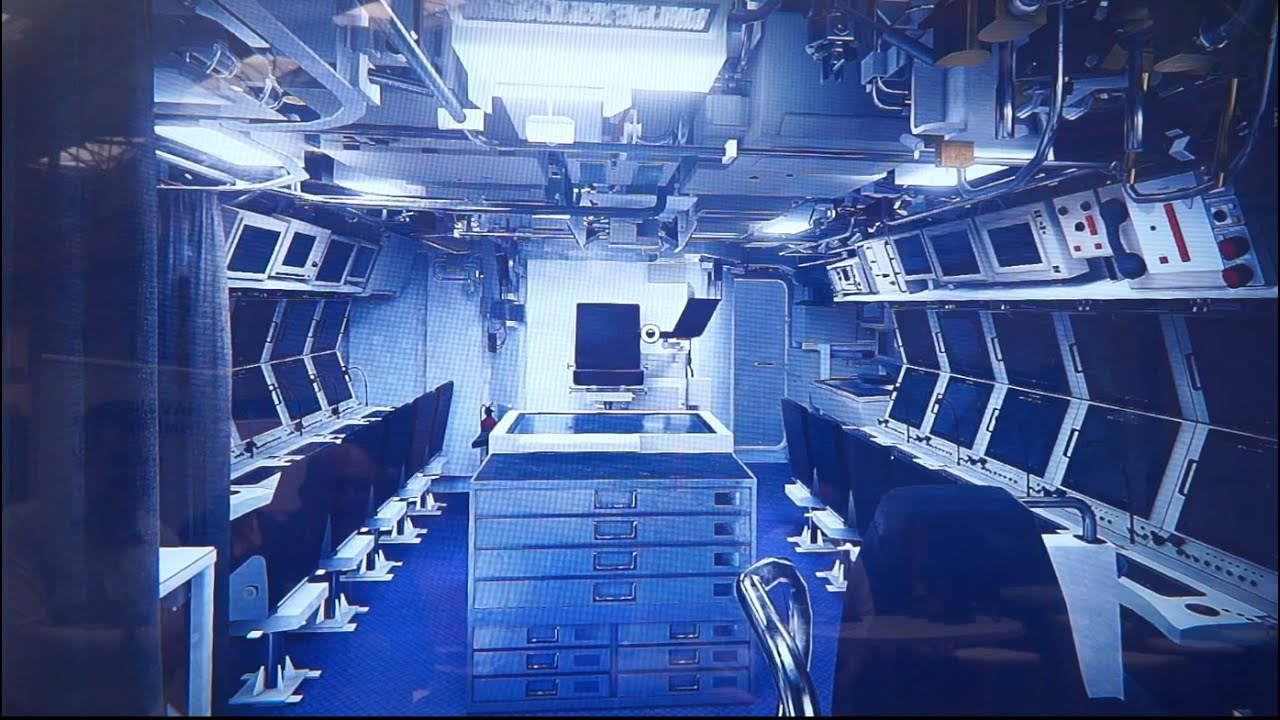The image depicts a technology-centric control room with a highly organized layout. Dominating the center of the room is a central table accompanied by a unit with numerous cabinet drawers, resembling a tool storage system. To the left and right sides of the room, rows of computer screens, arranged in a multi-level stack, occupy the walls. Each row features about five chairs that are mounted to the floor, all uniformly black with silver accents. Every chair is positioned in front of dual slanted monitors, creating an efficient workspace for each user. In the middle of the room sits a higher chair next to a laptop elevated on the central table. The room has a dark blue hue, accentuated by light blue and black tones, which contributes to its sleek, modern aesthetic. The ceiling features metal beams or rods, adding to the industrial feel, and there appears to be an opening or a light source at the top. A black curtain is visible peeking from the left side, and there are wires running across the ceiling, enhancing the high-tech atmosphere of the room.